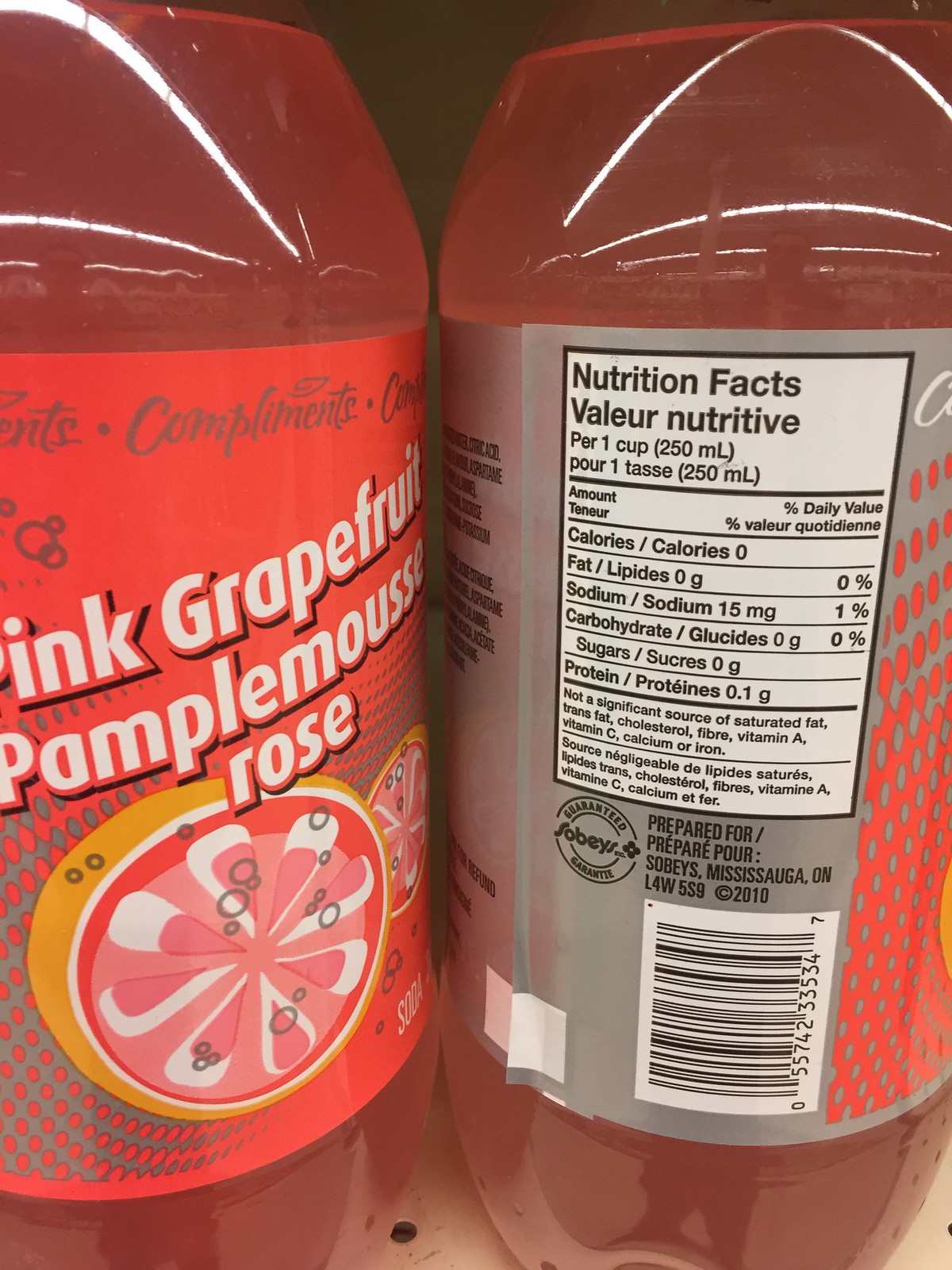This color photo captures two 2-liter bottles of pink grapefruit soda side by side, showcasing both the front and back labels. The vibrant pink liquid is visible through the clear plastic bottles, although their tops are cropped out of the frame. The bottle on the left features a bright orangey-pink front label adorned with the brand name "Compliments" and the text "Pink Grapefruit, Pomplemousse Rose." At the center of this label, an illustrated grapefruit is surrounded by a playful arrangement of bubbles.

The bottle on the right displays the back label, which predominantly contains nutritional facts on a grey background. This label is bilingual, with information presented in both English and French. Details include metrics on calories, fat, sodium, carbohydrates, sugars, and protein, revealing that the beverage is sugar-free. Further inspection reveals that the product is Canadian, distributed by Sobeys in Mississauga, Ontario. A barcode is also visible on this label, adding to the meticulous detailing of the bottle's design and information.